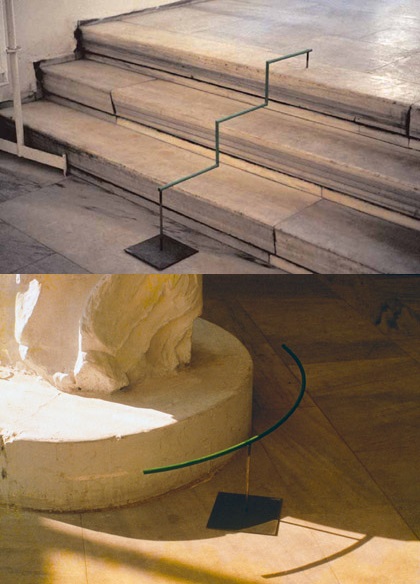This image features two distinct photographs, one above the other, potentially from a museum setting. The top photograph captures a staircase composed of gray tiles or bricks, featuring three steps. Midway through the staircase is a distinctive C-shaped green line structure, supported by black fin poles on both the top and bottom stairs. A white wall is visible in the top left corner. The bottom photograph depicts the base of a white plaster sculpture, partially visible with a circular green wire or stick encircling it, resting on a black pedestal frame. Sunlight illuminates the scene from the left, casting a shadow and adding depth to the base of the sculpture.